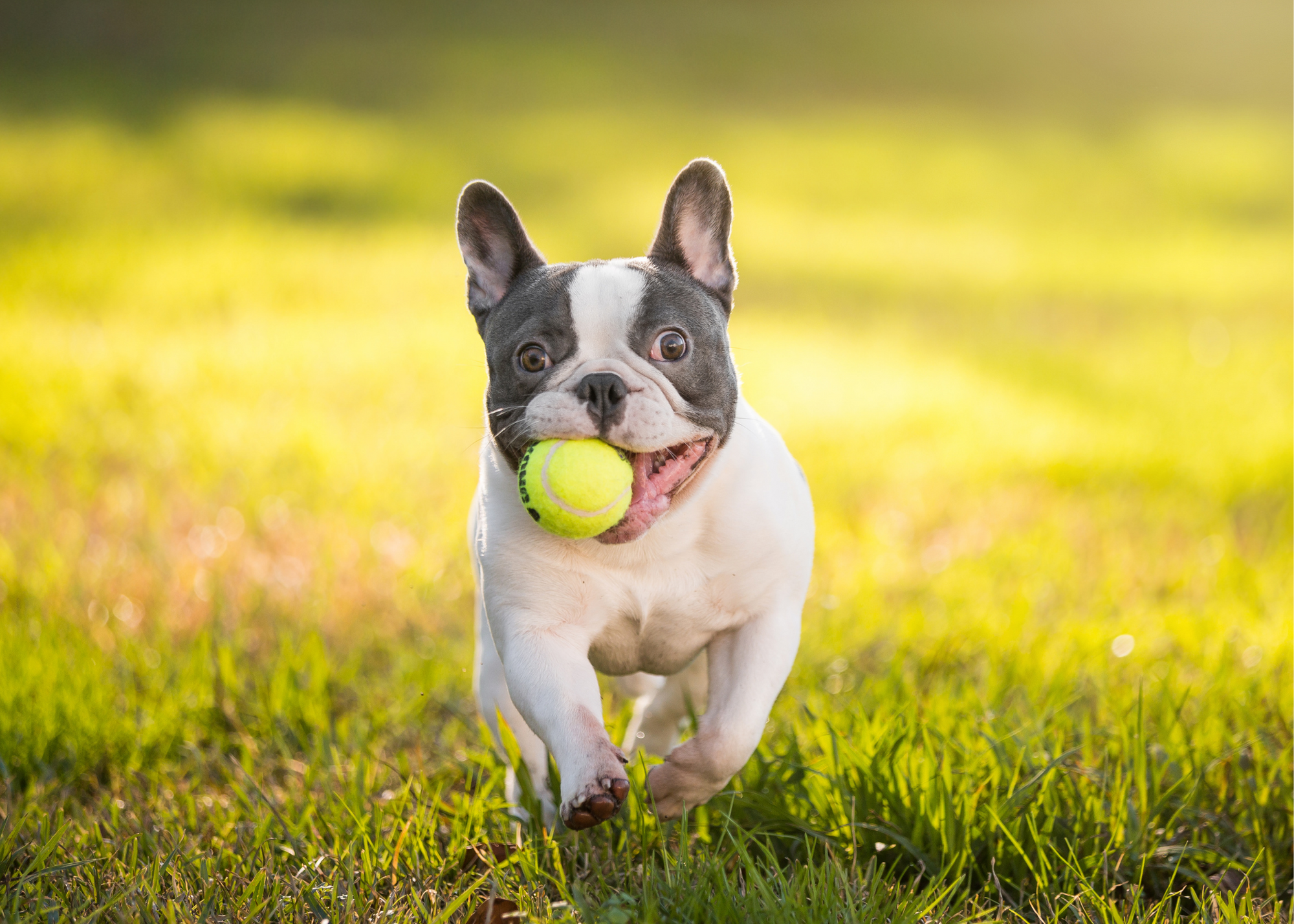In this detailed color photograph, a small, happy-looking dog, possibly a French Terrier or a breed similar to a Bull Terrier, is captured in mid-run, heading directly towards the camera. The image is taken from a low ground level, emphasizing the dog's eager movement. The dog's facial fur is a distinctive combination of dark gray (or black) around the cheeks, eyes, and ears, with a contrasting white strip running up the center of its face, forming a triangular shape. Its ears are large, standing erect with visible pink interiors. The body fur below the neck is cream-colored, and the dog is equipped with short, sturdy legs and broad paws.

The dog’s round eyes are alert, and it appears to be smiling, contributing to its excited expression as it holds a yellow tennis ball in its mouth. The grass in the foreground is several inches tall and dark green, sharply in focus, while the grass in the background gradually lightens in color and blurs out, suggesting a light source in the distance. This gradient effect enhances the sense of depth in the photograph, emphasizing the dog's joyful sprint through the grassy field. The overall style of the photograph is realistic and representational, capturing the lively moment in vivid detail.